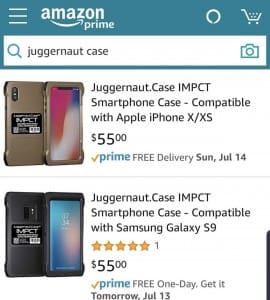The image depicts a mock-up of an Amazon Prime interface. At the very top, there's a dark blue border featuring a hamburger menu icon on the left and the Amazon Prime logo. On the right side of this border are a refresh button and a shopping cart icon. Below this border is a search bar containing a magnifying glass icon and the text, "juggernaut case," accompanied by a camera icon. 

The main section showcases two smartphone cases. The first is displayed both front and back, labeled as the "Juggernaut Case IMPCT Smartphone Case" compatible with Apple iPhone X/XS, priced at $55, with Prime free delivery slated for Sunday, July 14th.

Beneath a light gray horizontal divider, the second item is another smartphone case, also shown from the front and back. This case is described as the "Juggernaut Case IMPCT Smartphone Case" compatible with Samsung Galaxy S9. It has garnered five stars from one review, priced at $55, with Prime one-day delivery, arriving by tomorrow, July 13th.